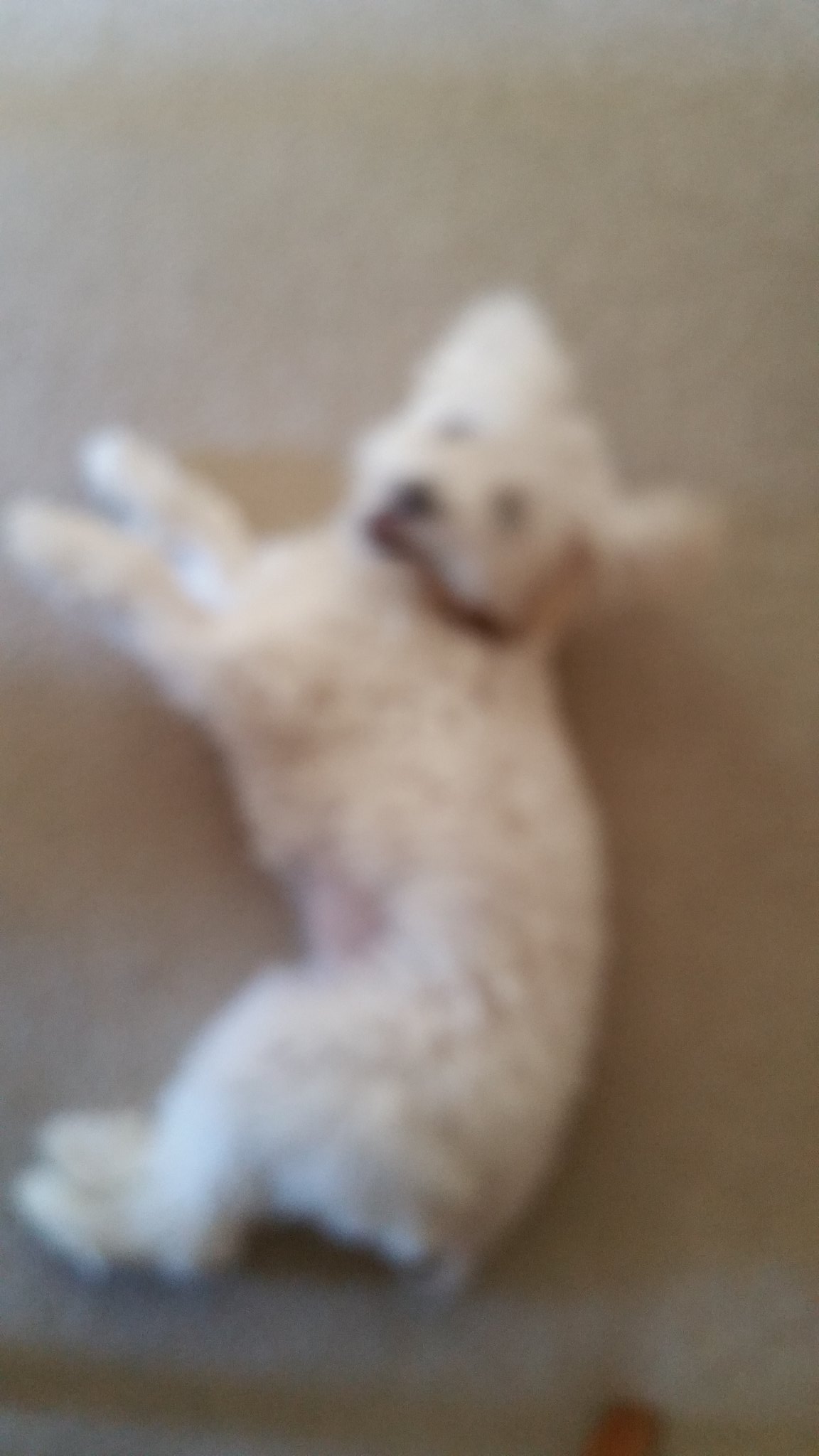In this image, we have a white, fluffy dog lying on the ground, though the picture is quite out of focus. Despite the blurriness, we can discern that this small dog, likely weighing less than 15 pounds, has a coat of soft, white, curly fur. The dog's features include small, dark eyes and a dark nose, although specific details are indistinct. The ears stand out as they are fairly pointy rather than floppy. The tail is not visible in the image, possibly due to the dog's small size, suggesting it might be a young puppy.